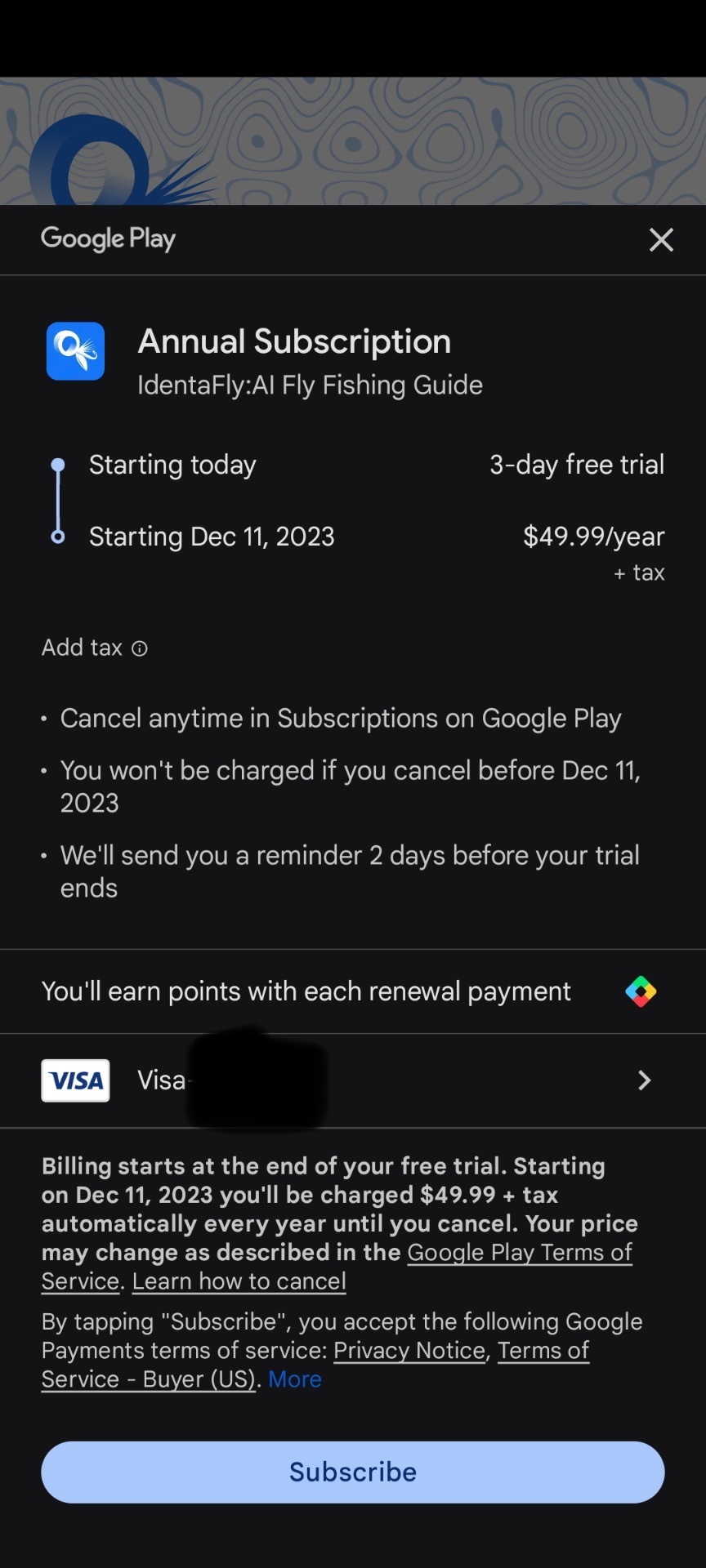The image shows a detailed subscription offer prompt from Google Play for the "Identify AI Fly-Fishing Guide." At the top of the screen, there is a heading that reads "Google Play" along with an X icon to close the window. 

The offer is for an annual subscription that begins with a three-day free trial starting on December 11th, 2023. After the trial period ends, the subscription costs $49.99 per year plus applicable taxes. Below the pricing details, three bullet points provide additional information:
1. You can cancel the subscription any time through Google Play without being charged if you cancel before December 11th, 2023.
2. A reminder will be sent to you two days before the trial period ends.
3. You will earn points with each renewal payment.

The bottom section specifies that billing will commence at the end of the free trial on December 11th, 2023, and you will be automatically charged $49.99 plus tax each year until you cancel. It notes that the subscription price may change in accordance with the Google Play terms of service. Finally, by tapping on the "Subscribe" button, you accept the Google payment terms of service, privacy notice, and relevant terms of service.